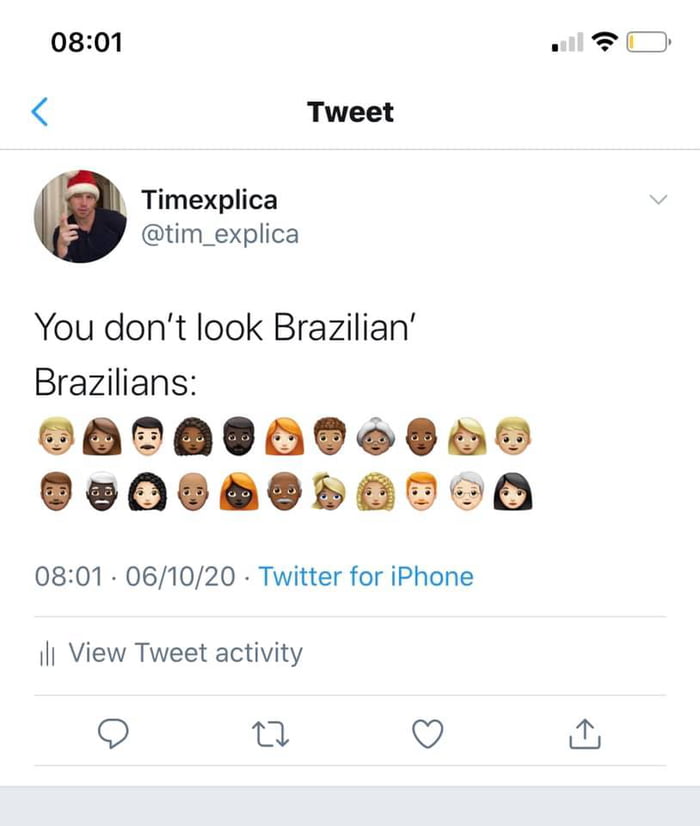A detailed screenshot from a mobile device displaying a Twitter interface on an all-white background. In the top left corner, the current time is shown in black as "8:01." On the top right, there are indicators for a weak Wi-Fi signal (one out of four bars), a connected Wi-Fi icon, and a nearly depleted battery icon.

Centered below, the word "Tweet" is prominently displayed in large, bold black letters. To the left of this is a blue back arrow.

Under a thin gray line, in the top-left corner, is a round profile picture of a young man wearing a black shirt and a Santa Claus hat. Next to the icon, to the right, are his name and handle: "Tim Explica" in black, with the username "@Tim_Explica" in gray beneath it. Over to the far right is a gray down arrow.

The tweet text reads: "You don't look Brazilian. Brazilians:" This is followed by two rows of diverse people emojis, totaling around 20, with variations in sex, hair color, and skin tone.

Below the tweet, in gray text, it notes the date and time "8:01 - 6/10/20", followed by "Twitter for iPhone" in blue. The final line of text in gray reads "View Tweet activity."

At the bottom of the screen are interactive icons: a speech bubble for replies, up and down arrows for retweets, a heart for likes, and an upward arrow above a U-shaped icon for sharing. The very bottom of the screenshot is bordered by a flat gray band running horizontally across the screen.